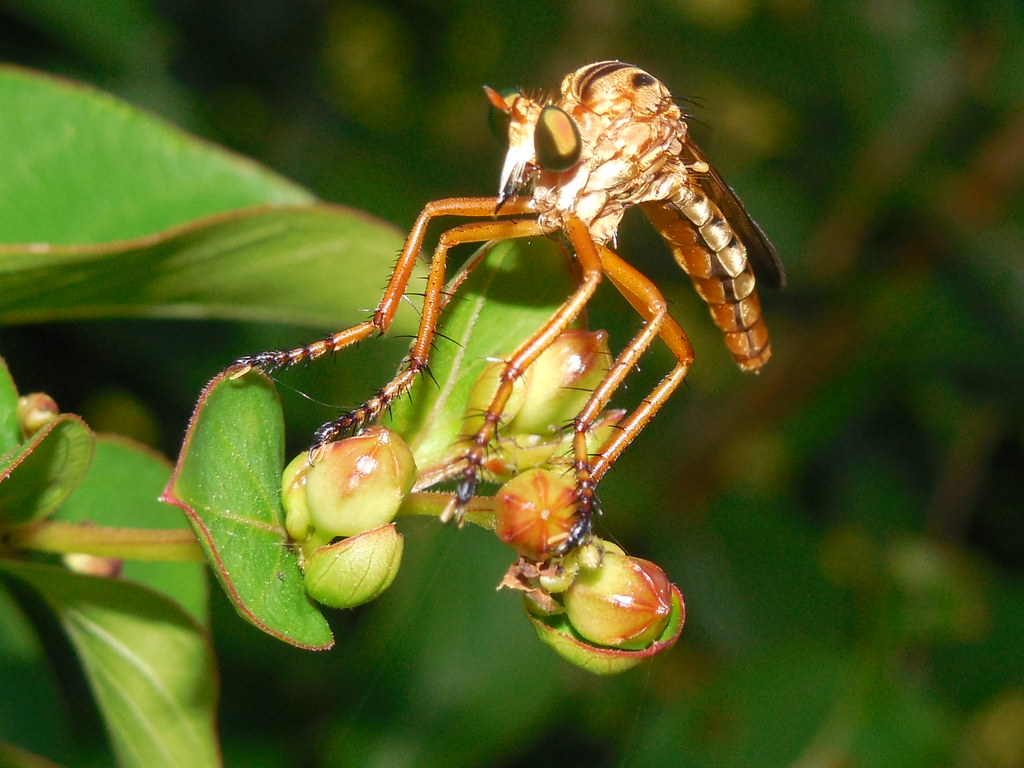This detailed color photograph, taken in landscape orientation, captures a close-up view of a young dragonfly perched on a cluster of lime green and red star-tipped berries. The dragonfly, centrally located in the image and facing the left, showcases an array of intricate features. It possesses oversized, black, and gold-highlighted eyes with a sharp, black-tipped mouth. The body of the dragonfly is segmented with beige scales and is predominantly brown, while its folded wings rest along its back. The dragonfly's six segmented legs, which are brown with black tips and adorned with hair-like structures, are seen gripping the plant leaves and berries. The background of the image is blurred, displaying patches of green, white, and brown, typical of photographic representational realism. On the left side of the frame, two or three large green leaves add to the natural setting.